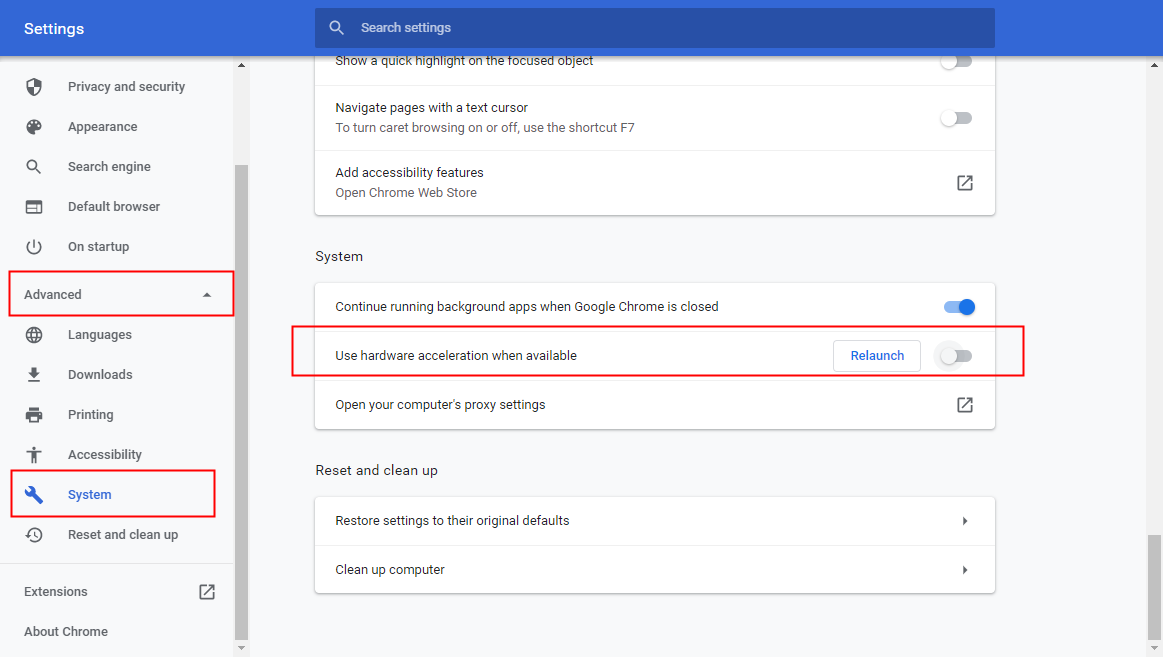The image showcases a settings menu on the left-hand side in a vertical layout. The title "Settings" is displayed in a blue bar that spans horizontally at the top of the menu, centered within this bar is a search bar labeled "Search settings." Below this bar, the settings menu is divided into three main sections, on a white background. The middle section, labeled "Advanced," is expanded, revealing several subsections: Languages, Downloads, Printing, Accessibility, System, and Reset and clean up. The "System" section is selected, which causes the main window on the right-hand side to display relevant options. This section contains three settings, one of which is "Use hardware acceleration when available," accompanied by a toggle switch that is currently off. A "Relaunch" button is also present within this section.